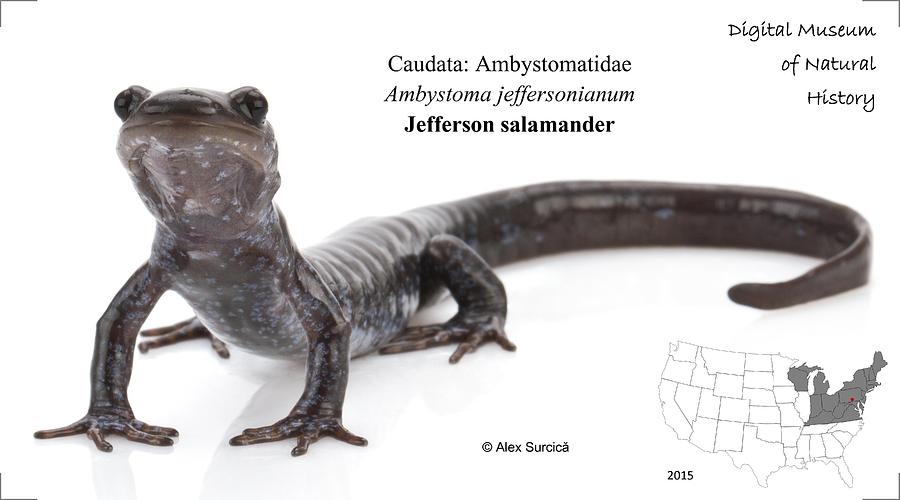This is a detailed photograph of a Jefferson's Salamander (Ambystoma jeffersonianum) prominently displayed in the center of the image. The salamander is a dark grey color with mottled lighter grey spots, and it’s positioned on its belly with its head raised, looking directly at the camera. The salamander's long tail curves gracefully to the right. The image is set against a white background and framed with black L-shaped corners that accentuate its rectangular format, roughly twice as wide as it is tall. Above the salamander, in bold black text, is its common name "Jefferson's Salamander," followed by its scientific classification: "Caudata Ambystomatidae Ambystoma jeffersonianum." To the right of the salamander and beneath its long tail, there's a black-and-white map of the contiguous United States, with portions of the Northeast, from Virginia up to Maine and parts of Michigan, shaded in grey to indicate its habitat range. In the upper right corner, it’s marked "Digital Museum of Natural History," and in the lower right corner, the date "2015" is listed above the copyright notice "© Alex Cersica."